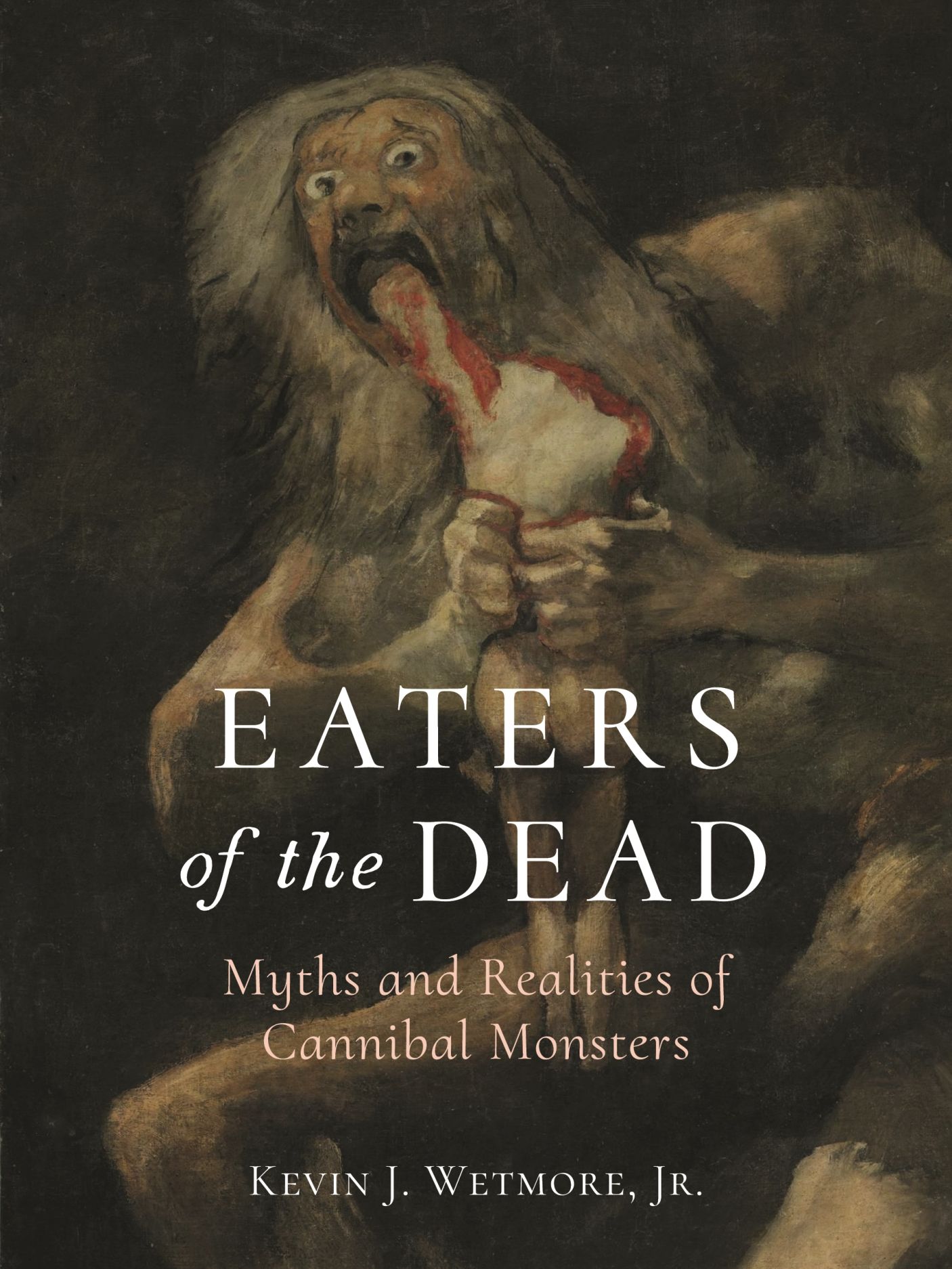The image features the cover of a book titled "Eaters of the Dead: Myths and Realities of Cannibal Monsters" by Kevin J. Wetmore, Jr. The cover artwork vividly depicts an ogre-like creature, reminiscent of a caveman or perhaps inspired by the mythological figure Kronos. This creature has wild, bulging eyes and stringy gray hair, which accentuate its ferocious appearance. 

With a dark, charcoal black background, the monstrous figure, with brown, hair-covered skin, stands out starkly. He is shown crouching, clutching in his hands the dismembered body parts—white and red flesh—that he ravenously consumes. The severed limbs, including a headless, armless torso, suggest the grisly act of cannibalism, possibly even the act of devouring a young child.

The book's title and the author’s name are prominently displayed in white, all-caps text centered from the middle down: "EATERS OF THE DEAD." Beneath this, in lowercase and smaller white letters, reads "myths and realities of cannibal monsters," followed by the author’s name, Kevin J. Wetmore, Jr. This cover effectively sets the tone for a deep exploration into the chilling myths and realities surrounding cannibalistic creatures in folklore and literature.